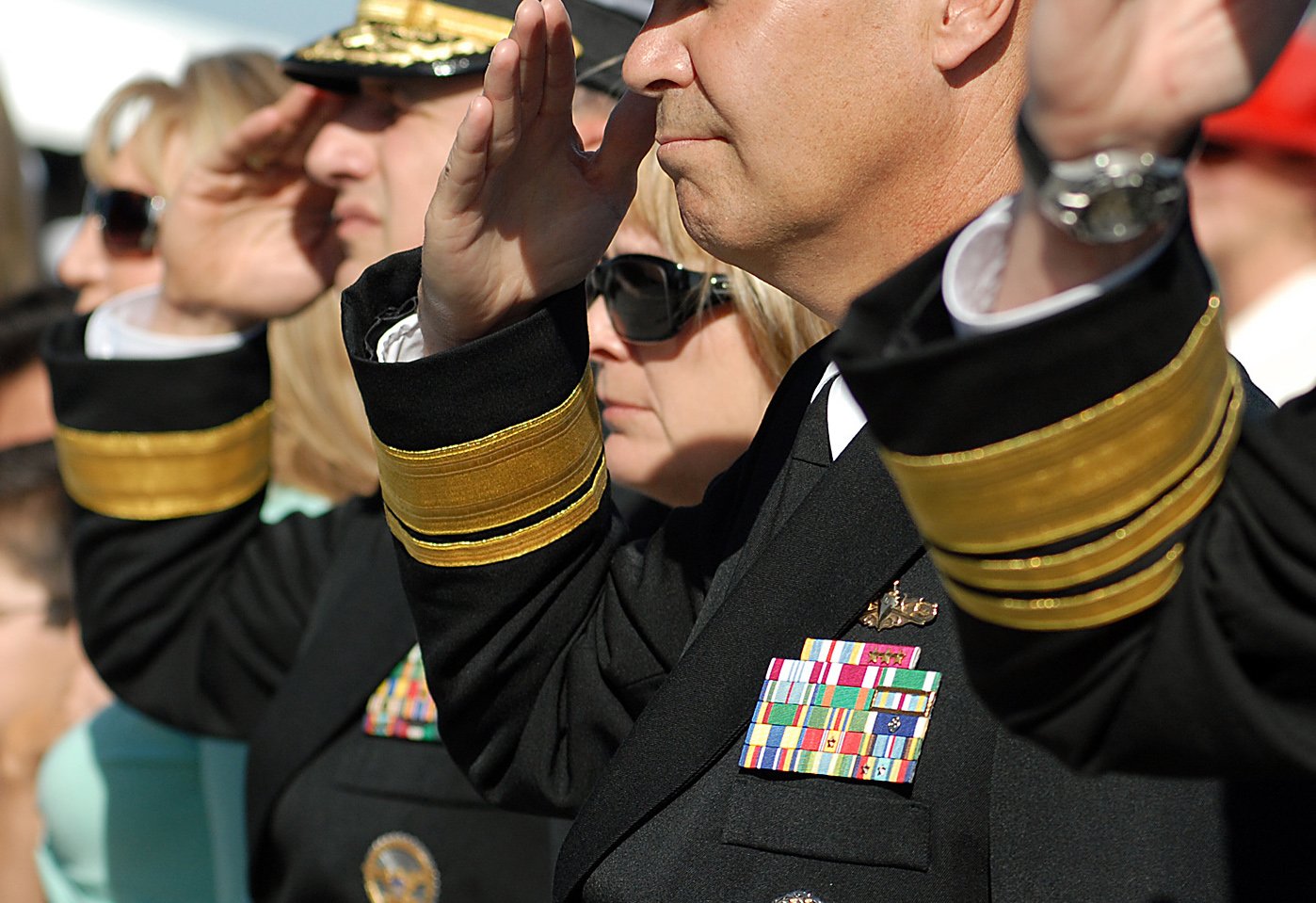This image captures a solemn military salute featuring four servicemen and women, each distinguishable through their detailed attire and position. The central figures consist of two men and two women, arranged from left to right. On the far left, a woman wearing sunglasses starts the lineup, followed by a man in a black and gold military uniform who is actively saluting. Next to him stands another woman in sunglasses. On the far right, another man in a similar black and gold uniform completes the group. This man’s uniform is adorned with various pins, including a black and gold one and a multicolored striped one, totaling 17 medals in all. The men are dressed in full military garb with black jackets, golden cufflinks, and white dress shirts underneath. Their expressions are serious, with the men's faces partially obscured but showing a concentrated, tense demeanor. The focus of the image is primarily on these servicemen, with the women likely being their counterparts. Additional, obscured figures linger on the outer edges of the frame, maintaining the image's central focus on the military subjects.